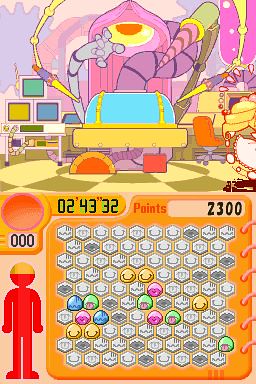Screenshot from a game showing intricate details: The top half of the image features a machine encased in a sleek blue cover with a prominent long purple pipe extending from it. The bottom half of the screenshot displays an orange panel filled with numerous hexagonal shapes. While some of these hexagons are color-filled, the majority remain in black and white. At the top of this panel, the word "Points" is displayed prominently, showing a score of 2300. Adjacent to this, on the left-hand side, a timer indicates that 2 minutes and 43 seconds are remaining.